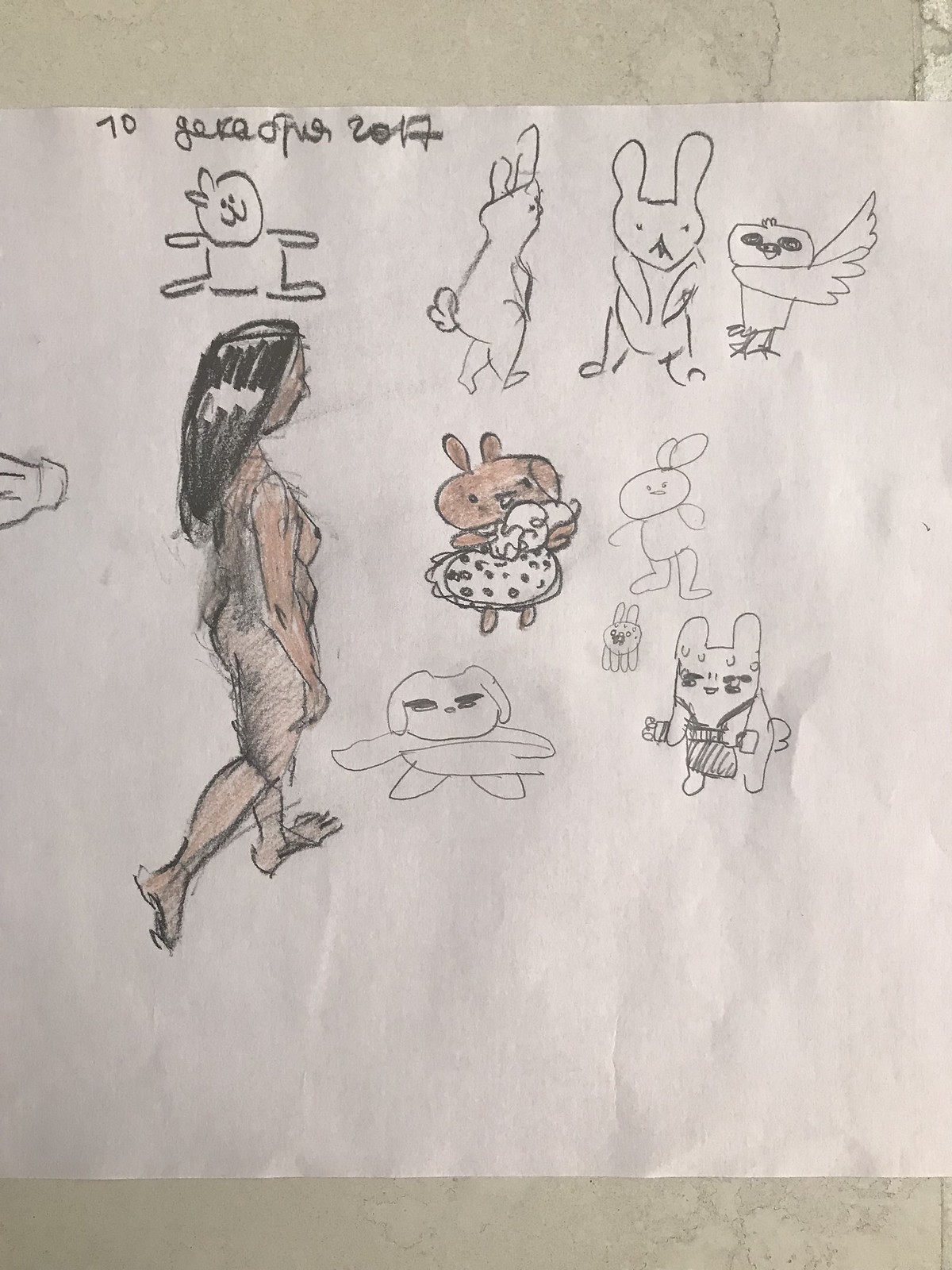The image showcases a crinkled, white sheet of paper set against a light tan surface, photographed as it lies horizontally. The paper contains an assortment of amateur pencil sketches, primarily of rabbits and other creatures, alongside a detailed depiction of a woman. In the top row, starting from the left, there is an outline of a rabbit with its head tilted to the left and legs splayed out. Next to it, another rabbit is drawn from a back-side angle, showing off its little puffy tail. Adjacent to this, a rabbit stands front-facing with rounded ears. Completing this row is an owl, depicted as if giving directions with its wings. The second row features a prominent figure: a nude woman, possibly with a cavewoman appearance, walking away and to the right. She has long dark hair with shiny highlights indicated by uncolored sections. Part of her right breast and side of her face are visible. To her right is a brownish-tan rabbit eating a pizza, and a loosely sketched rabbit with minimal details. Further down, another sequence includes a mother bunny holding a baby bunny, and an outlined bunny with a brown head. Scattered below are half-drawn and less detailed creatures. The overall composition is both whimsical and varied, showing a mix of completed and incomplete sketches.